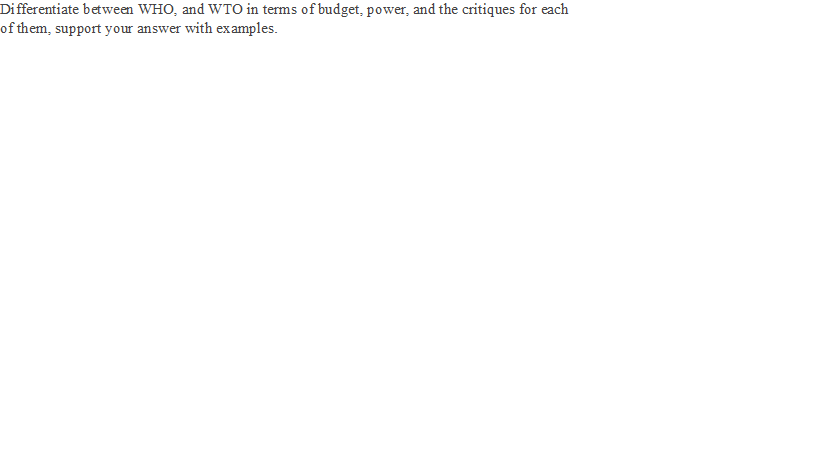An image with a stark white background features one sentence written in a classic serif font. The content of the sentence appears to be a question, likely from an exam. It reads: "Differentiate between WHO (World Health Organization) and WTO (World Trade Organization) in terms of budget, power, and critiques, supporting your answer with examples." This text is centered on the page, spanning one and a half lines with a carriage return after the W-H-O abbreviation and the full name in parentheses, followed by a comma and "WTO" on the first line. There is no additional content or imagery, creating a minimalistic and straightforward presentation.